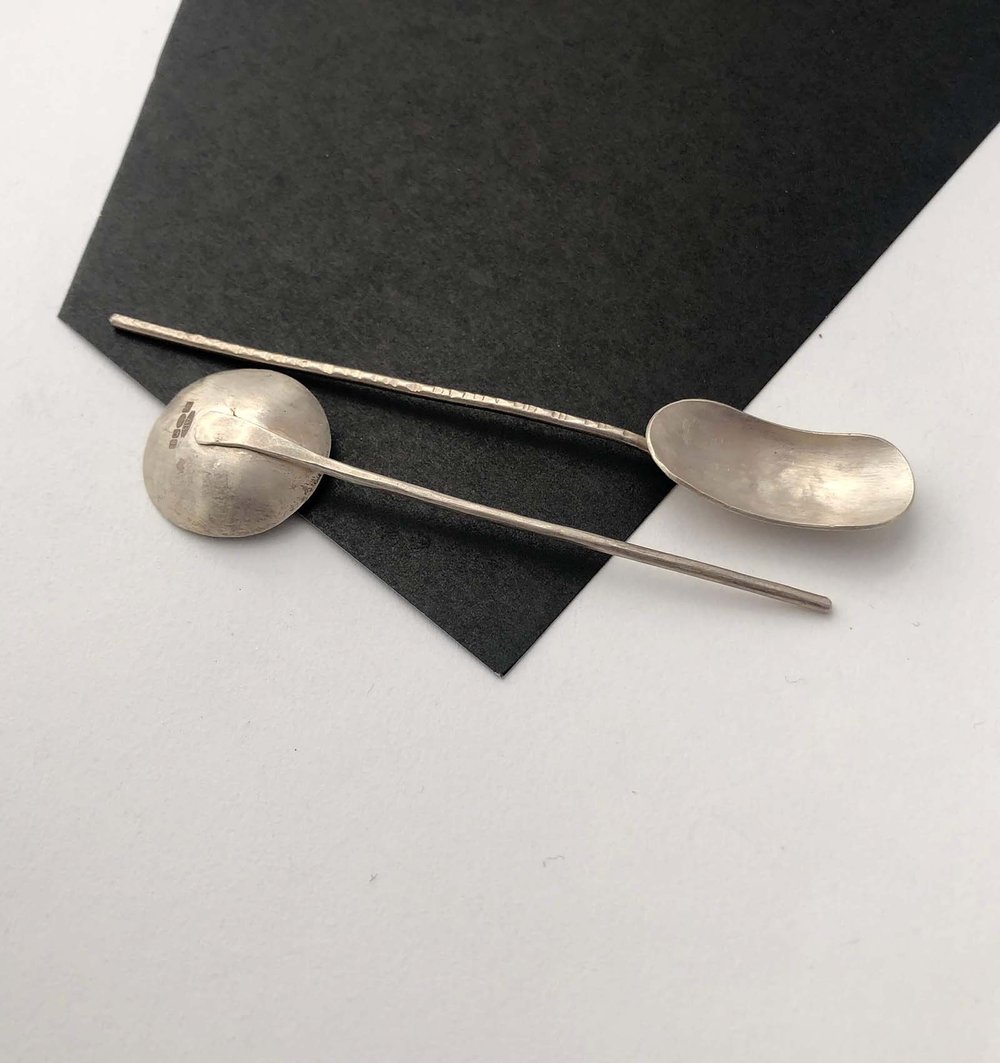This image, taken from above, showcases two likely silver utensils positioned against a white background. The utensils rest partially atop a dark black, irregularly shaped piece of paper that dominates approximately the top half of the frame. The top utensil, angled downward and facing the right, has an elongated, oval shape reminiscent of a jelly bean, with a thin handle and a scooped-forward design. The bottom utensil, facing the opposite direction, features a completely circular and shallow bowl-like structure - it is positioned upside down, revealing a stamped marking on its underside, which might indicate its silver material. Both utensils have a light silver hue, reflecting a dull yet noticeable sheen.